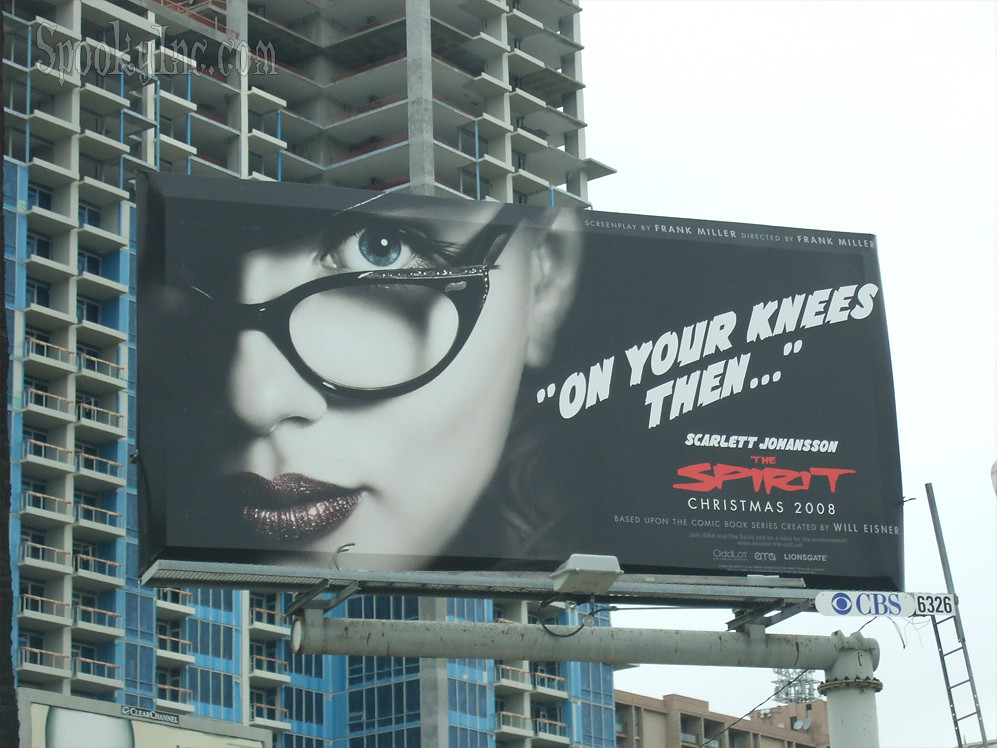This daytime color photograph prominently features a large billboard mounted on a metal pole, complete with a ladder on its right-hand side. The billboard has a striking black background, with the left side showcasing a close-up image of Scarlett Johansson. She is wearing black cat-eye glasses and dark red lipstick, with one green eye visible, exuding a serious expression as she looks out at the viewer. The right side of the billboard contains text in white and red; in white letters, it reads "On Your Knees Then" followed by "Scarlett Johansson," and in bold red letters, it says "The Spirit," with "Christmas 2008" written just below. Below the billboard, there is a light fixture aimed upwards to illuminate the ad at night and a small plaque reading "CBS 6326". In the background, we can see a large high-rise building under construction, featuring gray floors and blue scaffolding.